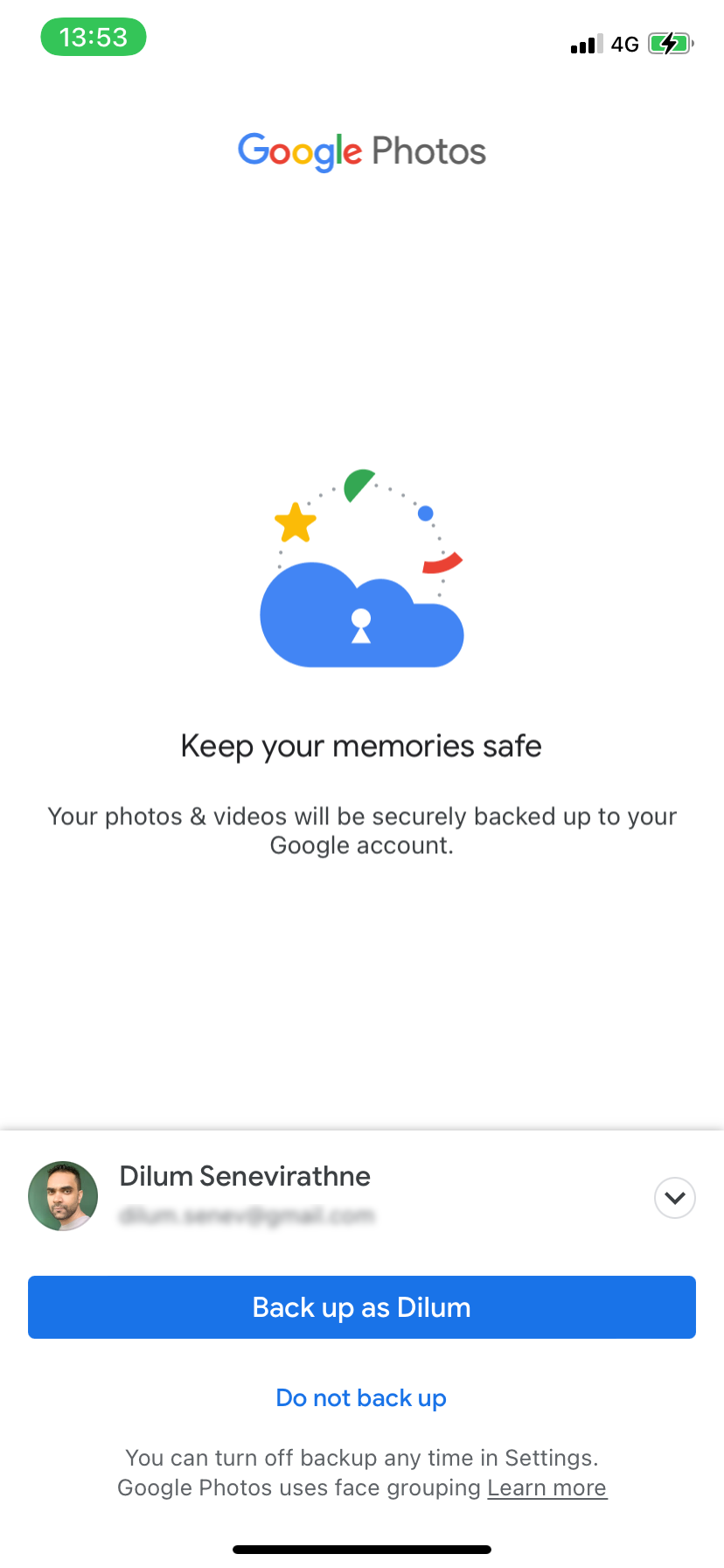The image is a screenshot from a cell phone. At the top left, a green button displays the time as "13:53" in white font. To the right of the time, the cell phone reception icon shows three bars and indicates "4G," followed by a fully charged battery icon. Centered below these icons, the text "Google Photos" is prominently displayed.

Beneath this heading, there is a blue cloud icon with a white keyhole symbol inside it. Encircling the cloud are several graphical elements: a star, a half circle, a small circle, and a partial edge of another circle, creating a dynamic visual.

Below this iconography, the text "Keep your memories safe" is featured, followed by an explanation: "Your photos and videos will be securely backed up to your Google account."

Towards the bottom of the image, there is a space and then a circular profile picture.